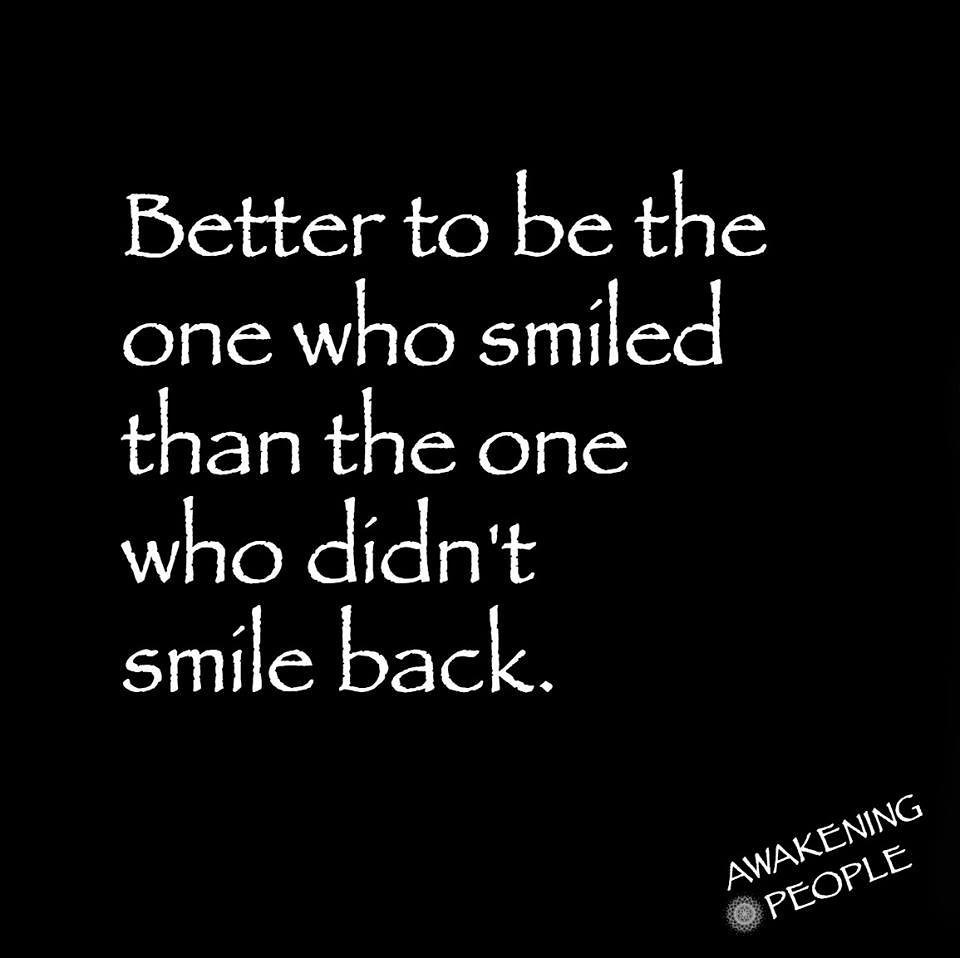This image features a black background with a distressed-looking white sans serif font displaying the quote: "Better to be the one who smiled than the one who didn't smile back." The quote is centered and split into five lines for emphasis. In the bottom right corner, there is smaller text in uppercase reading "AWAKENING PEOPLE," accompanied by a small, detailed mandala-like circle. The mandala appears to be the logo of "AWAKENING PEOPLE," the apparent creator of the image. The contrast between the white text and the black background makes the message clear and striking.